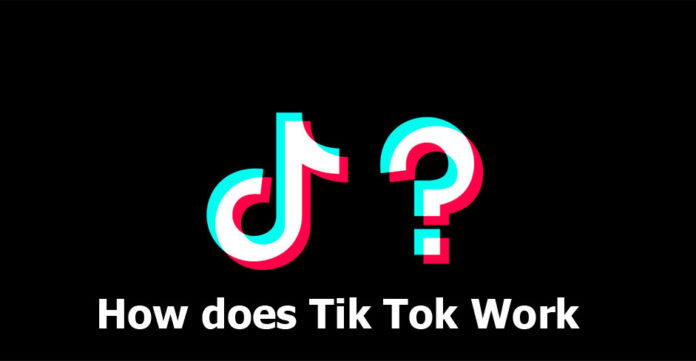This digital image, formatted as a horizontal rectangle with approximate dimensions of 16x9, features a minimalist logo accompanied by text. At the center of the frame are two distinct graphical elements. On the left, an eighth note is depicted in two overlapping colors: a red version slightly shifted up and to the left overlapping with a bright blue version. The intersection of these colors creates a white area, giving it a three-dimensional effect reminiscent of 3D movie visuals. 

To the right of this, there is a similarly styled graphic, this time featuring a question mark. The question mark consists of two overlapping versions as well: a pink one positioned down and to the right, and a blue one shifted up and to the left, with their intersection also forming a white section, enhancing the 3D effect.

Below these graphics, a line of white, sans serif text reads "How does TikTok work" with specific capitalization: the 'H' in 'How,' the 'T's in 'TikTok,' and the 'W' in 'work' are all capitalized. The text is evenly spaced with no additional punctuation, and the spacing between words is uniform.